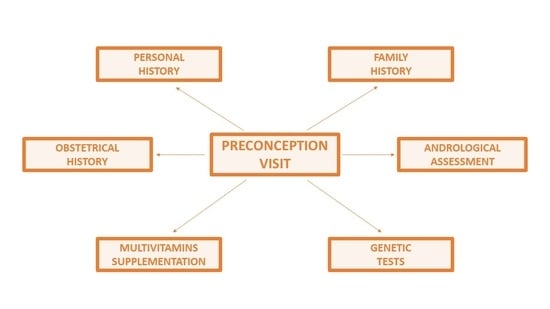The image depicts a detailed color diagram resembling a mind map, set against a white background. At its center, there is a larger rectangular box outlined in orange with the text "pre-conception visit." Surrounding this central box, there are six smaller orange-outlined rectangles, each connected to the central box by arrows. These rectangles are arranged in a circular pattern, with three on the left and three on the right.

Starting from the top left and moving clockwise, the boxes read:
1. Personal History - Top left.
2. Family History - Top right.
3. Andrological Assessment - Right.
4. Genetic Tests - Bottom right.
5. Multivitamin Supplementation - Bottom left.
6. Obstetrical History - Left.

Each rectangle features text in a brownish-orange color. The diagram's design employs peach or dark pink hues for the rectangles, which adds a visually cohesive element to the layout. The central "pre-conception visit" box serves as the core focus, with thin arrows pointing outwards to each of the surrounding rectangles.